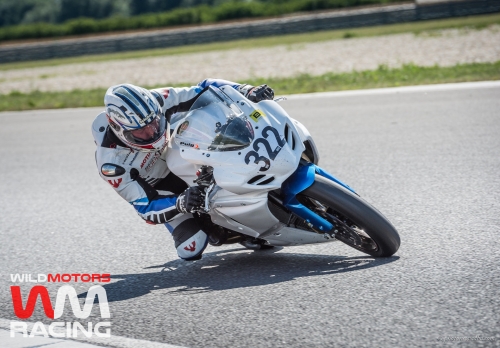This is a detailed color photograph capturing a motocross racer mid-turn on a blue and silver motorcycle, prominently displaying the number 322 on the front. The person and motorcycle are dramatically leaned to the right, almost grazing the gray asphalt, indicative of a high-speed maneuver on a racetrack. The racer is clad in full motorcycle gear: a blue and white long-sleeved shirt with some black accents, white pants, black and white knee pads, thick black gloves, and a multi-colored helmet in silver, black, and blue with a clear visor. 

The background features a strip of green grass, extending towards what appears to be a dirt or walking track, and further back, a cement barrier and additional green foliage. The lower left corner of the photograph contains a red and white logo reading "Wild Motors" with "WM Racing" beneath it, suggesting this is a promotional or professional racing image. The overall scene is bathed in sunlight, highlighting the action and intensity of the sport.